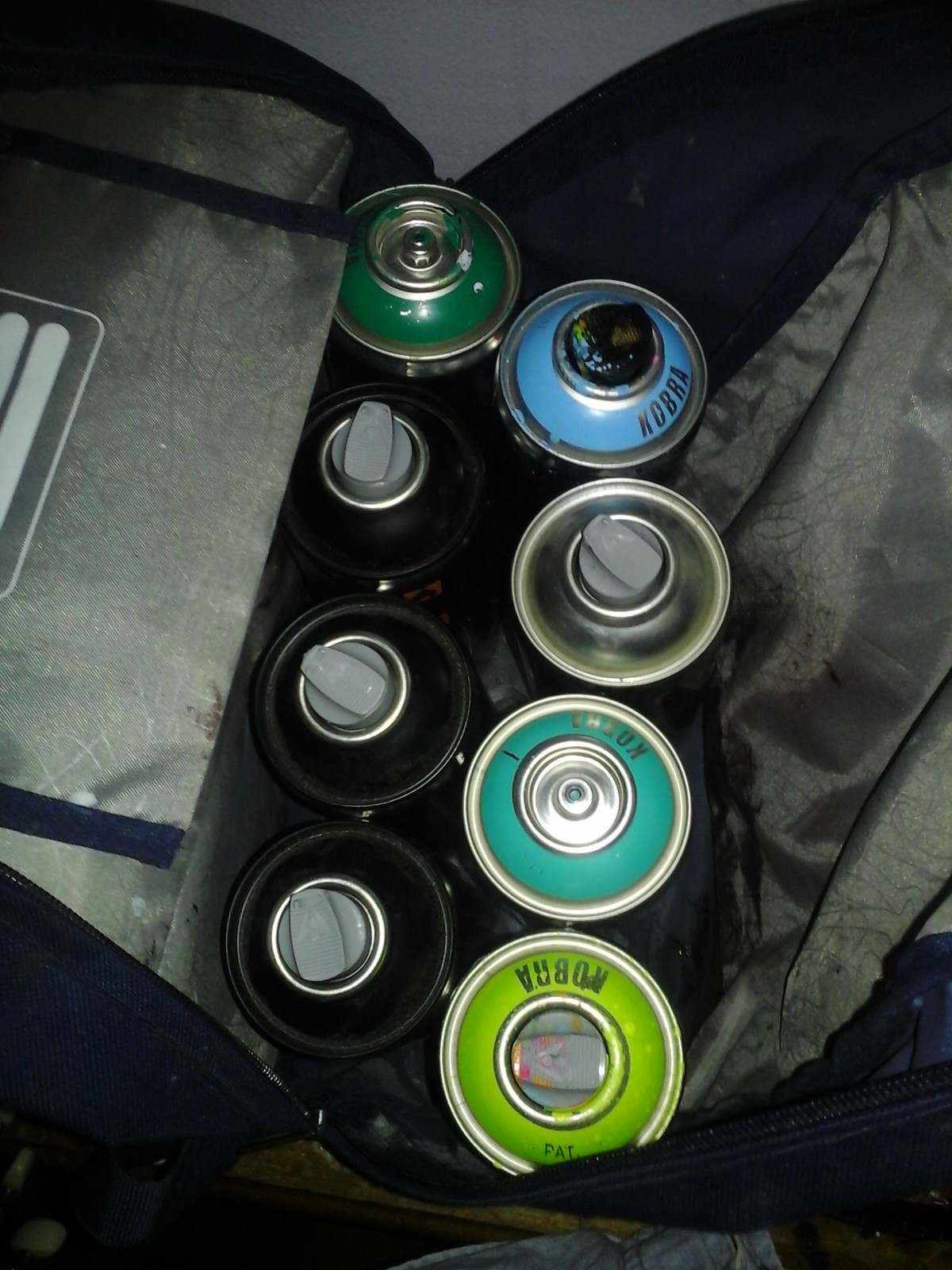The image displays a close-up view into an open black bag with a silvery gray fabric lining. Inside the bag, there are eight spray cans arranged in two rows of four. The tops of the cans are visible and come in various colors. On the right side, the spray can tops are colored light green, aquamarine, gray, and light blue. On the left side, the tops are dark green, black, black, and black. Of the eight cans, five have gray spray nozzles, and one has a black nozzle; notably, the aquamarine and dark green cans are missing their spray nozzles. One can even has some pink splatter on it, suggesting they might be used for paint. The configuration and details hint that these are indeed paint spray cans stored inside the bag.